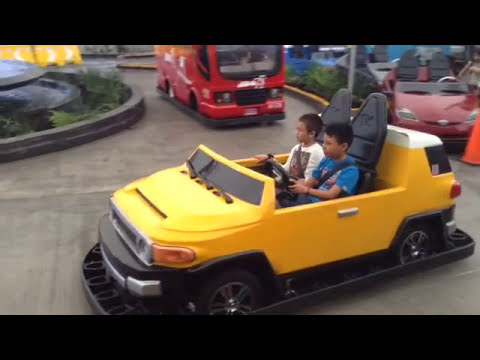The image shows a daytime outdoor scene at a go-kart track, framed by horizontal black bands at the top and bottom. Centrally featured is a small yellow SUV-style go-kart Hummer with tall seats and a small black windshield, designed to fit two occupants. Seated inside are two young boys with brown skin and black hair, the driver wearing a blue short-sleeved t-shirt with blue jeans, and the passenger in a white long-sleeved shirt with a dark green graphic on the front. The yellow go-kart has black bumpers around its base. In the background, there are other small bumper cars, including a notable red bus and a red convertible, as well as an orange traffic cone. The track is paved with a round curb visible on both the upper left and right sides of the image.